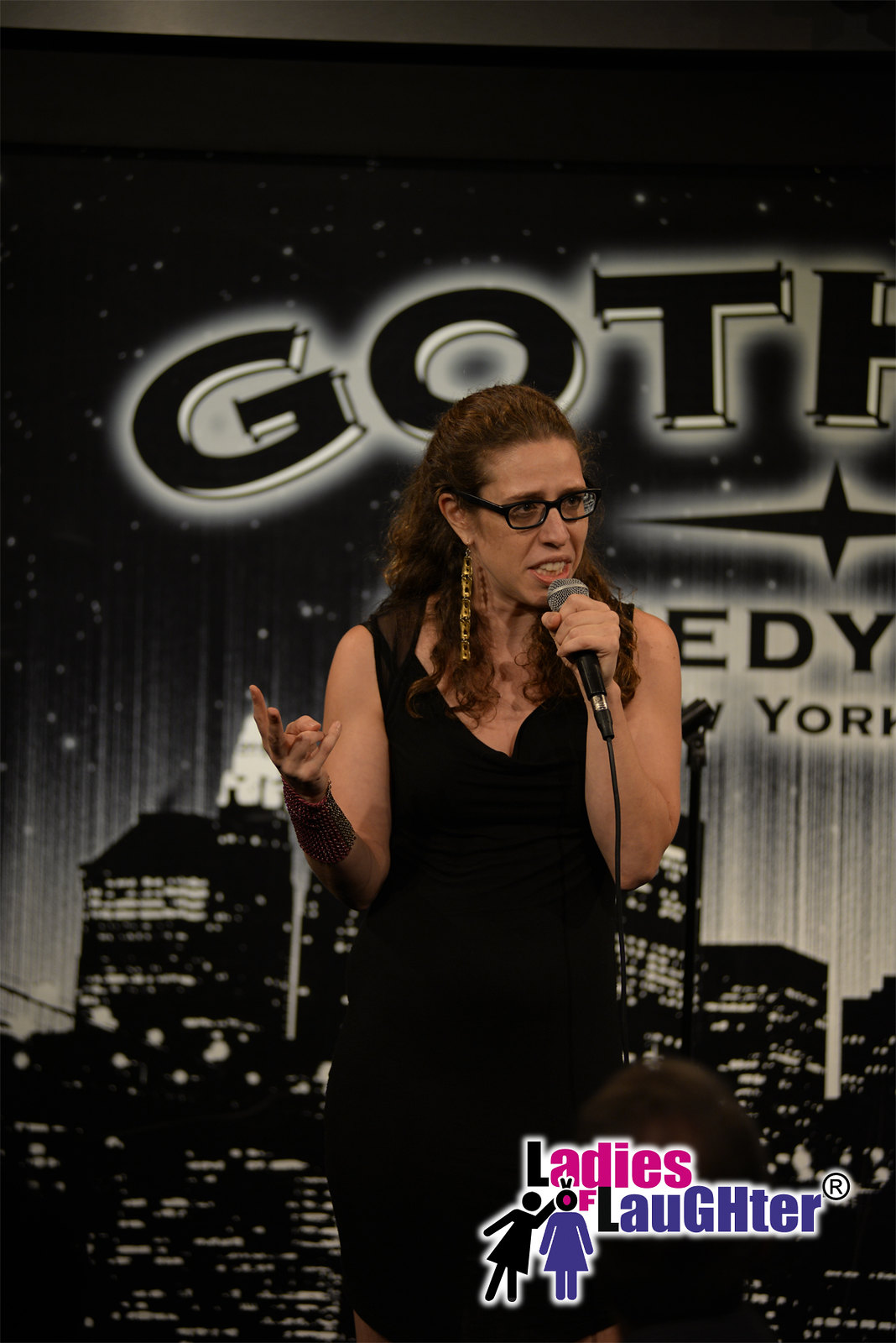The image captures a woman on a stage, presumably performing stand-up comedy, signaled by the "Ladies of Laughter" watermark logo at the bottom right of the photo. The logo features a palette of black, pink, and blue, complete with a trademark symbol. The woman is dressed in a sleeveless black dress, adorned with a long bracelet on her left wrist and a gold-colored, lengthy earring. She holds a wired microphone in her left hand and makes a ‘V’ or number two sign with her right hand, suggesting she might be counting or emphasizing a point. She has curly brunette hair cascading over her shoulder, wears eyeglasses, and has a light complexion. The background features a black-and-white city skyline with stars and glow lines, providing a nighttime urban atmosphere. The top-left portion of the background partially displays the text “Goth,” potentially hinting at “Gotham,” and below it, there is a car manufacturer’s logo likely connected to the venue. The scene is characterized by typical stage lighting and composition, further emphasizing the performance setting.